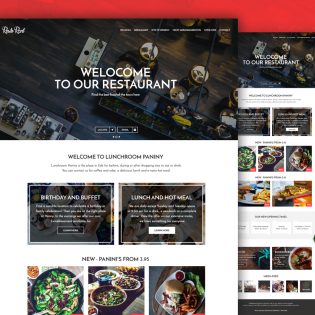A screenshot of a web page for "Lunchroom Panini" restaurant. At the top of the page, there is a prominent typo where "Welcome" is incorrectly spelled as "Wellocome." The background of the top image features an aerial photograph of the restaurant's interior. Below this, the text "Welcome to Lunchroom Panini" greets visitors.

The web page is segmented into sections with two rectangular boxes underneath the greeting text. The box on the left is labeled "Birthday and Buffet," while the box on the right is labeled "Lunch and Hot Meal." Further down, a banner advertises "New Paninis from $1.95."

There are three photographs of dishes offered at the restaurant displayed at the bottom of the page. The first image on the left depicts a large salad bowl filled with various colorful leaves and strips of what appears to be chicken or another type of white meat. The second image displays a burger served on a plate alongside some chips.